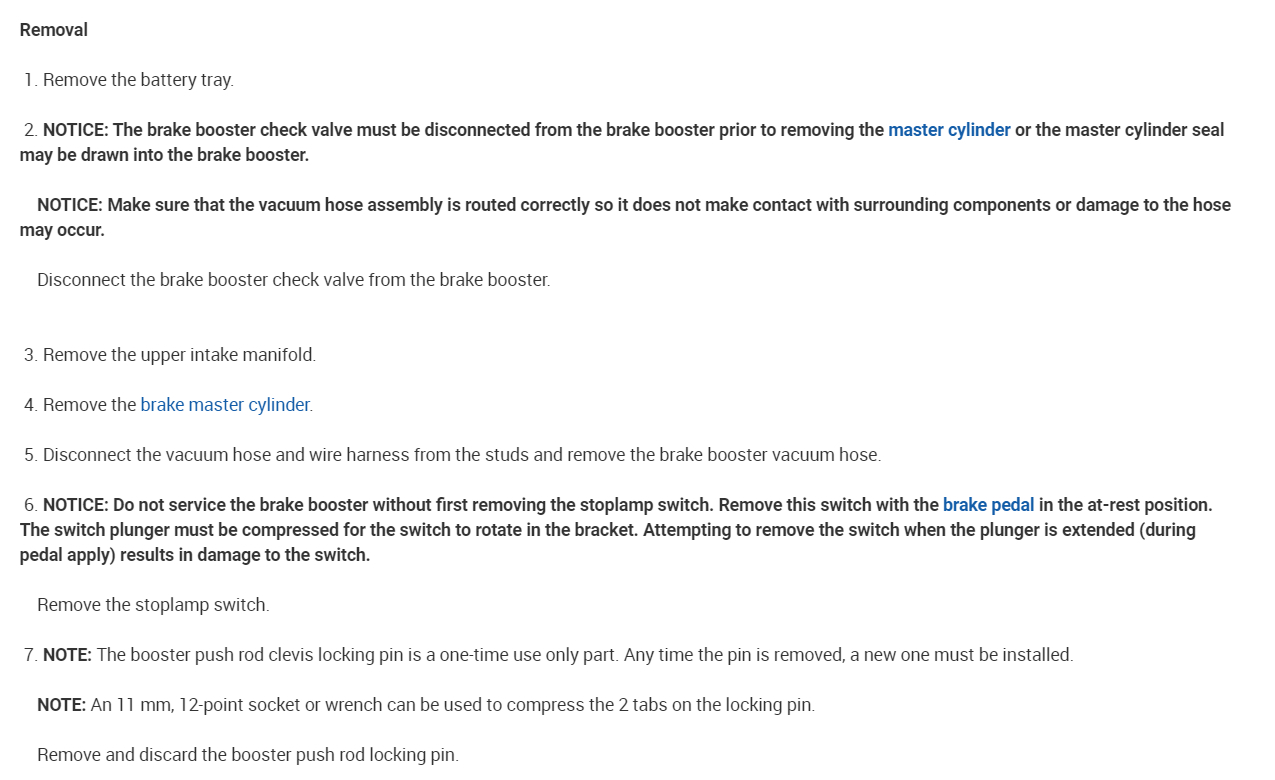**Descriptive Caption for the Image:**

The screenshot showcases a webpage with a predominantly white background and black text. The document appears to be an instructional guide for the removal of a brake system component. 

In the upper left corner, the word "REMOVAL" is prominently displayed in bold black text. The instructions are enumerated as follows:
1. Remove the battery tray.
2. **NOTICE:** The **brake booster check valve** must be disconnected from the brake booster prior to removing the master cylinder, to avoid drawing the master cylinder seal into the brake booster. **NOTICE:** Ensure the vacuum hose assembly is correctly routed to prevent contact with surrounding components, which could result in hose damage.
3. Disconnect the brake booster check valve from the brake booster.
4. Remove the brake master cylinder.
5. Disconnect the vacuum hose and wire harness from the studs and remove the brake booster vacuum hose.
6. **NOTICE:** Do not service the brake booster without first removing the stop lamp switch. Remove the switch with the brake pedal in the at-rest position, as the switch plunger must be compressed for proper removal. Attempting to remove the switch with the plunger extended could result in damage to the switch. Remove the stop lamp switch.
7. **NOTE:** The booster push rod clevis locking pin is a single-use part. A new pin must be installed if the old one is removed. **NOTE:** Using an 11 mm 12-point socket or wrench, compress the tabs on the locking pin to remove and discard it. 

Notably, some key terms, like "master cylinder," appear in blue, emphasizing their importance. "NOTICE" and "NOTE" sections are highlighted in bold and capital letters to grab the reader’s attention effectively.